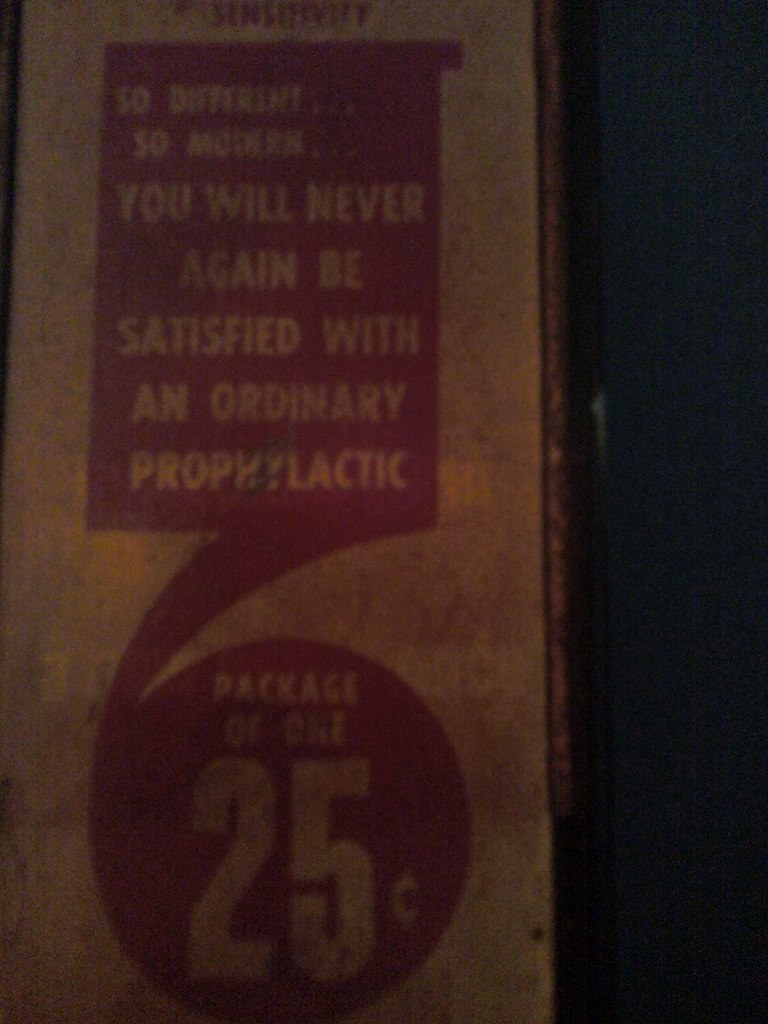This image features an underexposed, darkened photograph of a vintage wooden advertisement sign with visible aging and wear. The sign has a red painted background with white lettering that reads, "So different you will never again be satisfied with an ordinary prophylactic." There is a notable red box at the top of the sign, though the text within is partly cut off and difficult to discern. A red line extends from the bottom-right corner of this box, forming a red circle that prominently displays the price, "Package of 1.25 cents," with the "25" significantly larger. The sign appears to be the only object in the dimly lit photo, which lacks additional detail due to its dark and blurry nature.